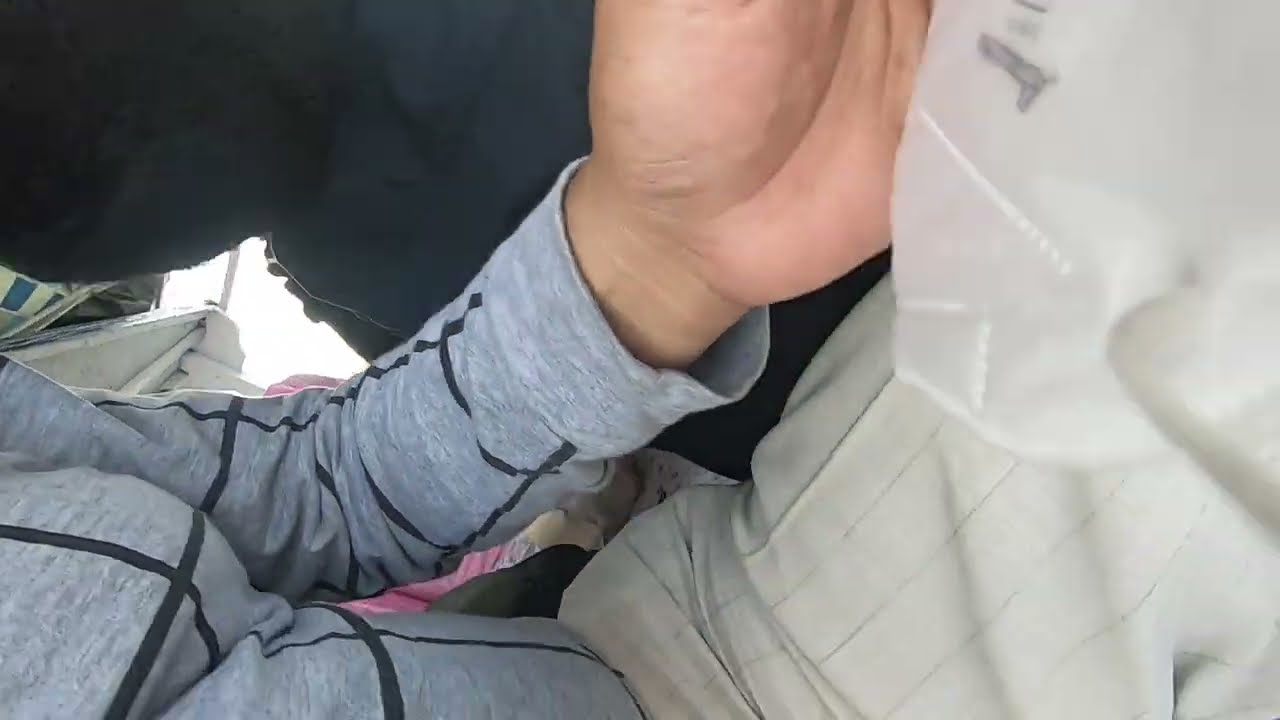This full-color, vertically rectangular photograph has been taken sideways. It mainly captures a person's left hand and wrist, potentially slightly showing parts of their chest, belly, and leg. The person is wearing a long-sleeve gray shirt adorned with a pattern of black lines forming squares. Their pleated pants, which might be tan or white, cover part of their lap. The individual appears to be holding a white object with black markings, which resembles an N95 mask. There's noticeable daylight coming through what looks like a window in the background. Additionally, there's a presence of medical equipment and perhaps a person in a black jacket or pink attire, indicating that the setting could be a hospital. The composition implies that the picture might have been taken by the person themselves using their right hand.